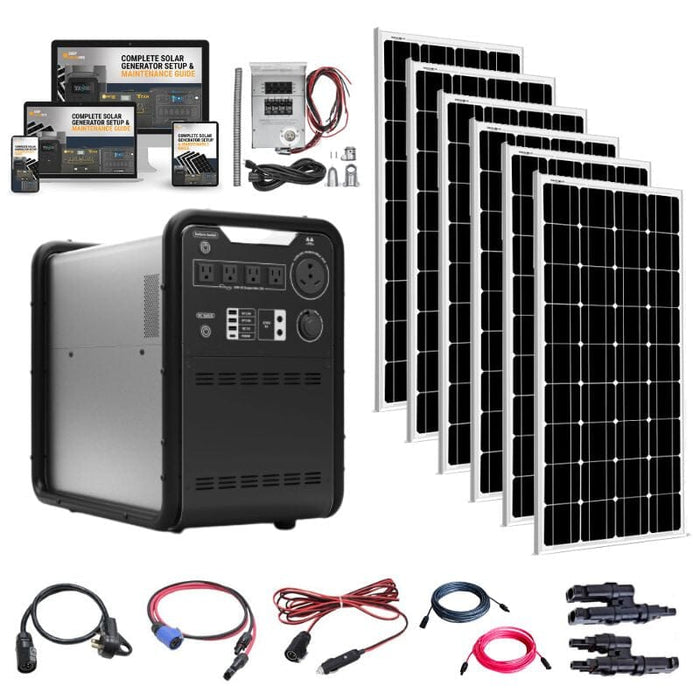The image features a complete solar generator setup with accompanying maintenance guide. Dominating the right side, six black and white solar panels are stacked in a cascading manner, each panel consisting of a 4x9 grid of 36 cells. The frames of the panels are white, contrasting with the black cells. To the left, a rectangular generator with black ends and a silver body is prominently displayed. Surrounding the generator, several screens show the digital instruction manual, accessible via various devices such as a phone, tablet, TV, and laptop.

At the bottom of the image, five smaller pictures showcase the necessary cables and plugs for the setup. These include black cords, black and red cords, and various plugs, laid out in an organized line. Additionally, some black components that resemble handles or mounting hardware for the solar panels are visible. Coiled cables and an additional small electrical box with wires are also present, illustrating the array of components required for the complete solar energy system.